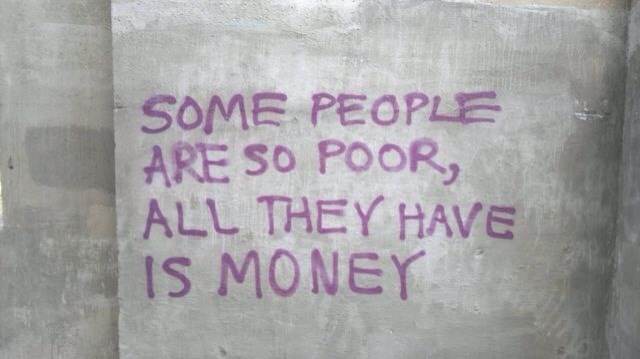This is a photo of a gray concrete wall with a horizontally oriented rectangular dark section on the left side. The wall features streaks of lighter gray, giving it a textured, painted appearance. In the center, large purple capital letters are neatly and evenly spaced, displaying the phrase, "Some people are so poor, all they have is money." The text is arranged across four lines: the first line reads "Some people," the second line says "Are so poor," the third line contains "All they have," and the fourth line concludes with "Is money." The wall and text are the sole elements in the photograph, emphasizing the profound message conveyed by the neatly executed graffiti.